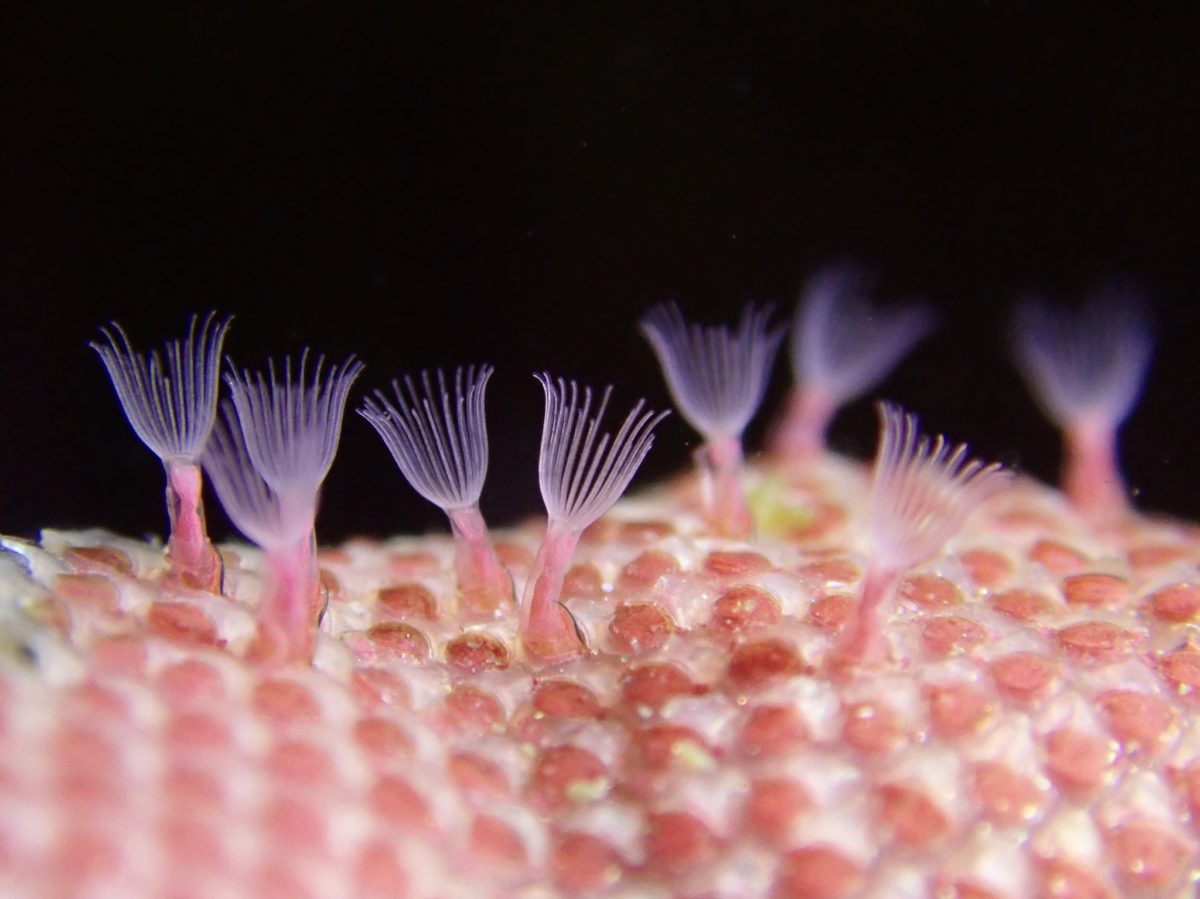The image features a close-up view of a microscopic marine creature, appearing like tiny sea anemones amidst a backdrop of black. These creatures are observed growing from red, dot-like pods scattered across the bottom half of the frame, which resembles a bumpy skin-like mat. There are nine of these anemone-like entities, organized so that five are located on the left side and four on the right. Each creature has a semi-transparent, pinkish trunk that emanates from the red pods, adorned with delicate, very thin, white tentacles forming a circular shape reminiscent of flowers before they fully bloom. The pink stems are relatively thicker compared to the ultra-thin white lines that spiral gracefully around them, reaching varying heights. Overall, the image offers a strikingly detailed and organized view of this unique underwater or cellular scene illuminated meticulously against the pitch-black background.